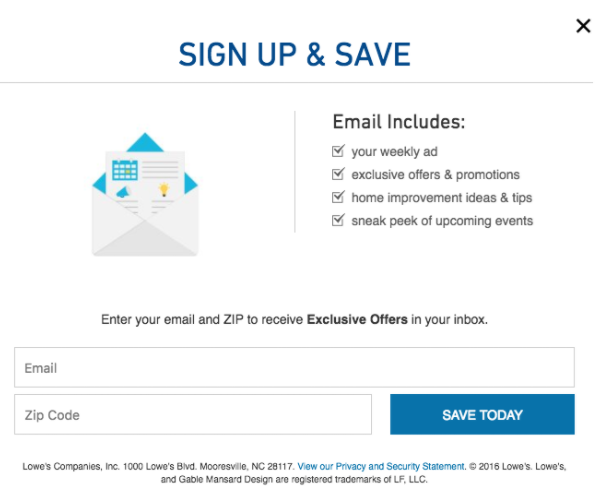This image is a screenshot of a sign-up page from a website, most likely from Lowe's. The page prominently features an email sign-up form aimed at offering promotional content and updates to subscribers. On the left side of the page, there is a large graphic of an envelope with a letter emerging from it, emphasizing email communication. 

The main text reads "Sign Up and Save" and elaborates on the benefits of subscribing via email, which include:
- Weekly ads
- Exclusive offers and promotions
- Home improvement ideas and tips
- Sneak peeks of upcoming events

Below this information, there are input boxes for users to enter their email addresses and ZIP codes. The email input box is clearly labeled "Email," and the ZIP code input box is labeled "ZIP code." To the right of the ZIP code box is a blue rectangular button labeled "Save Today" in white text.

At the bottom of the screenshot, company details are listed: "Lowe's Companies, Inc., 1000 Lowe's Boulevard, Mooresville, NC 28117." There is also a prompt to "View our policy and security statement." The page footer marks the content as © 2016 Lowe's and notes that both "Lowe's" and the "Gabby Mansard design" are registered trademarks of LF, LLC.

In summary, this is a detailed sign-up page for Lowe's aimed at encouraging customers to subscribe for special offers and updates.